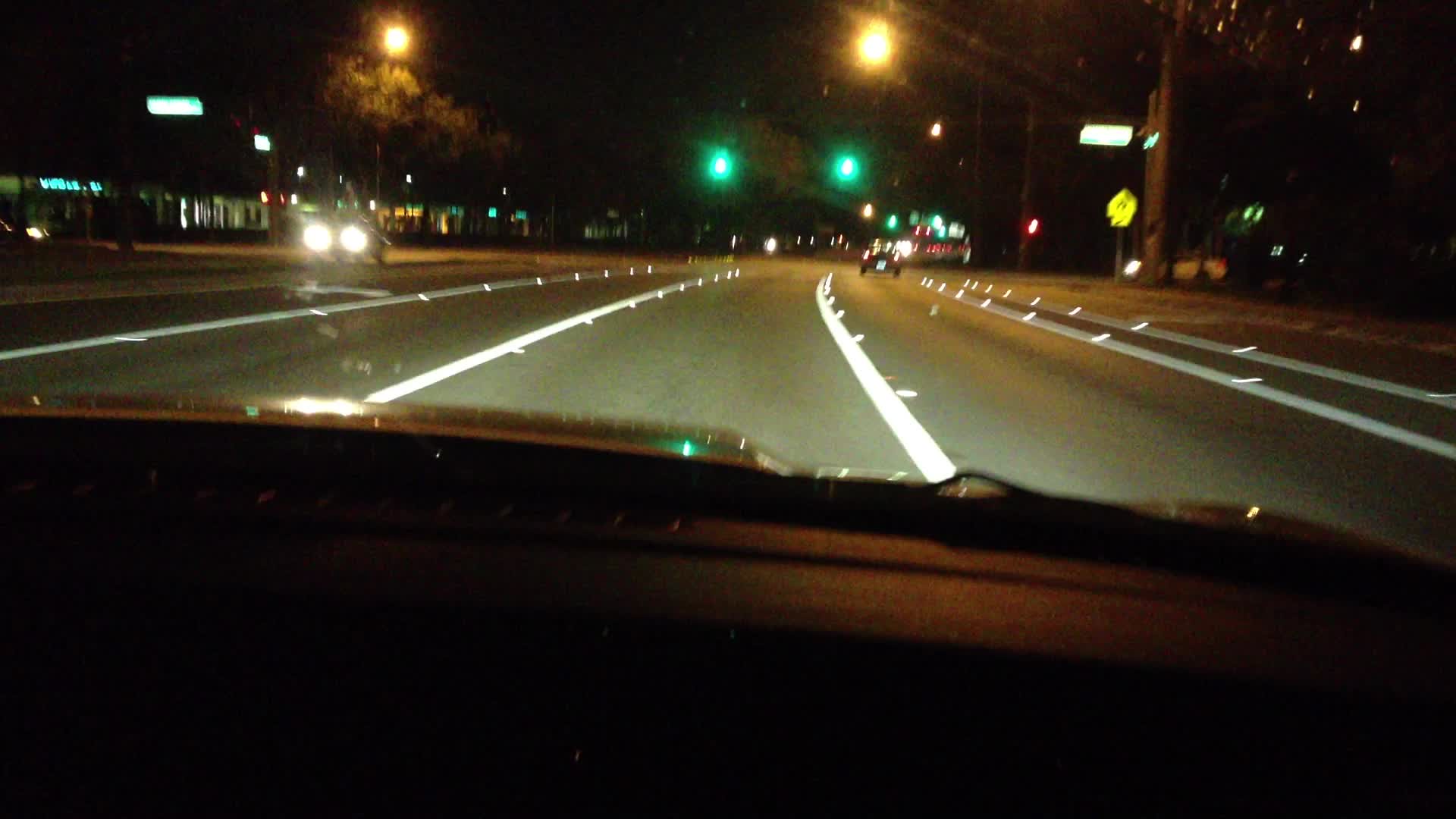The photo captures the interior of a vehicle driving at night. The bottom half of the image is dominated by the dark dashboard, shrouded in near-complete darkness. The top half reveals the vehicle's position in what appears to be a left-turn lane, illuminated primarily by oncoming traffic. A car approaches from the opposite direction, its headlights piercing through the night.

Ahead, the scene is lit by various streetlights, creating a bright backdrop. On the right side of the image, an indistinct street sign is visible followed closely by a yellow school crossing sign. The vehicle is nearing an intersection governed by two vivid green traffic lights, signaling the path forward. To the left, there are several stores, though their details are blurred, adding to the nocturnal atmosphere of the scene.